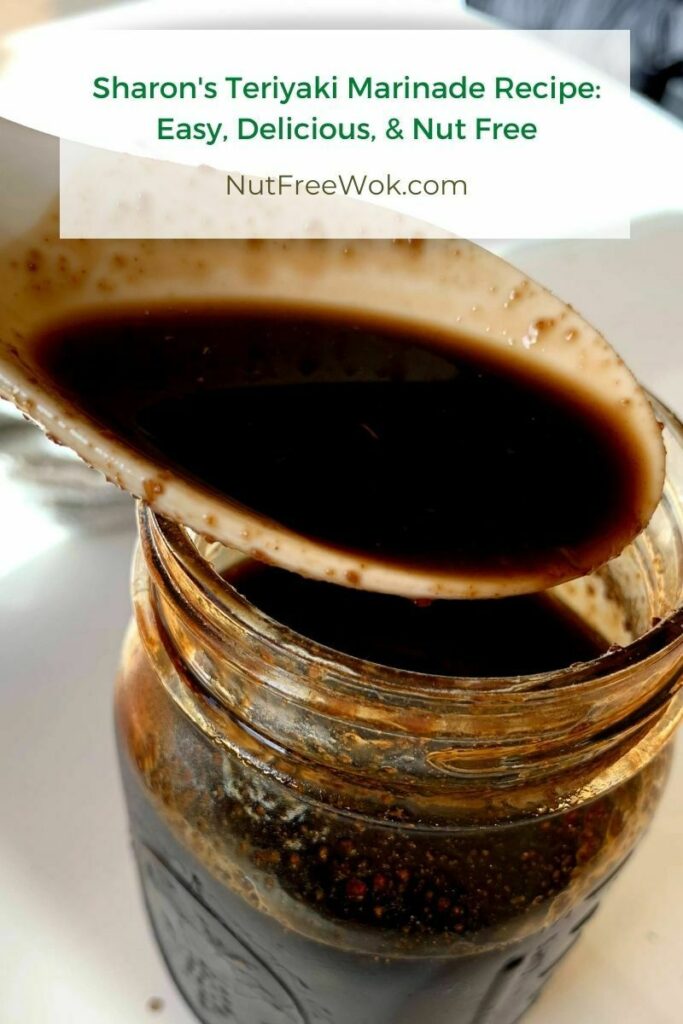The image is a close-up of a glass mason jar filled with a dark, black-brown liquid featuring small specks of red, identified as Sharon's Teriyaki Marinade. The jar is approximately 80% full and rests on a white counter. Hovering above the jar is a white oriental-style spoon holding a portion of the marinade, with the spoon's contents clearly visible. At the top of the photograph, text in a green font reads "Sharon's Teriyaki Marinade Recipe: Easy, delicious, and nut-free," followed by black text stating "nutfreewalk.com." The photograph, taken from an overhead angle, focuses on the jar and the spoon, while the background is blurred to emphasize the product.